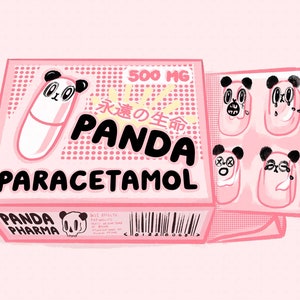The image showcases an animated depiction of a pink medicine box labeled "Panda Paracetamol" in bold black font. The box is open, revealing a blister pack of four individual pills. Each pill humorously features a panda's face, complete with eyes, nose, and ears. The top right corner of the box prominently displays "500 MG," while beneath this in Japanese characters and in large print, the word "Panda" is diagonally written across the box. Below this, "Paracetamol" is clearly marked. The sides of the box feature the logo "Panda Pharma," adorned with a panda with a skull head design. A pale pink background accentuates the overall whimsical theme, with additional designs of dots and Asian writing adorning the top of the box. The box and its contents appear upright, adding to the organized and cohesive presentation.